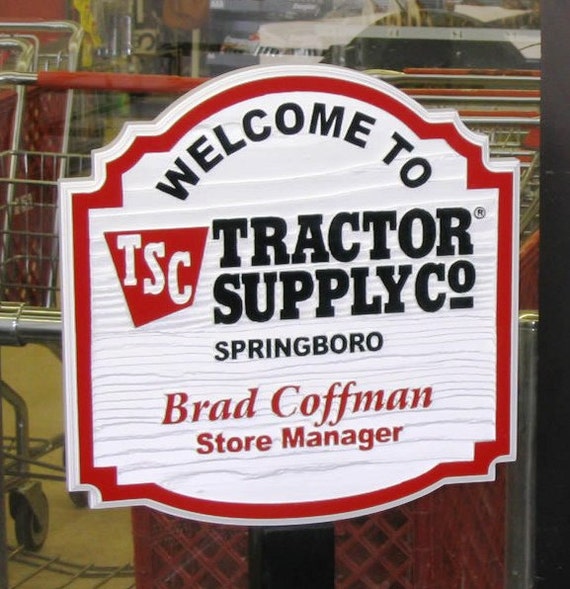This photograph features a detailed view of a white wooden sign with a red border, prominently displayed in a window of what appears to be a Tractor Supply Co. store. The sign is rectangular, with a trapezoid-shaped TSC logo in white on a red background on the left-hand side. The text on the sign is formatted as follows: "Welcome to" is written at the top in black text, followed by "Tractor Supply Co" and "Springboro," also in black text. Below that, "Brad Kaufman, Store Manager" is written in red text. The sign's surroundings include several shopping carts visible behind it, hinting at its location near the store's entrance. In the background, there are miscellaneous objects indicative of an indoor retail setting, and the sign itself is supported by a black base at the bottom. The image is closely cropped, focusing primarily on the sign and the immediate area around it.